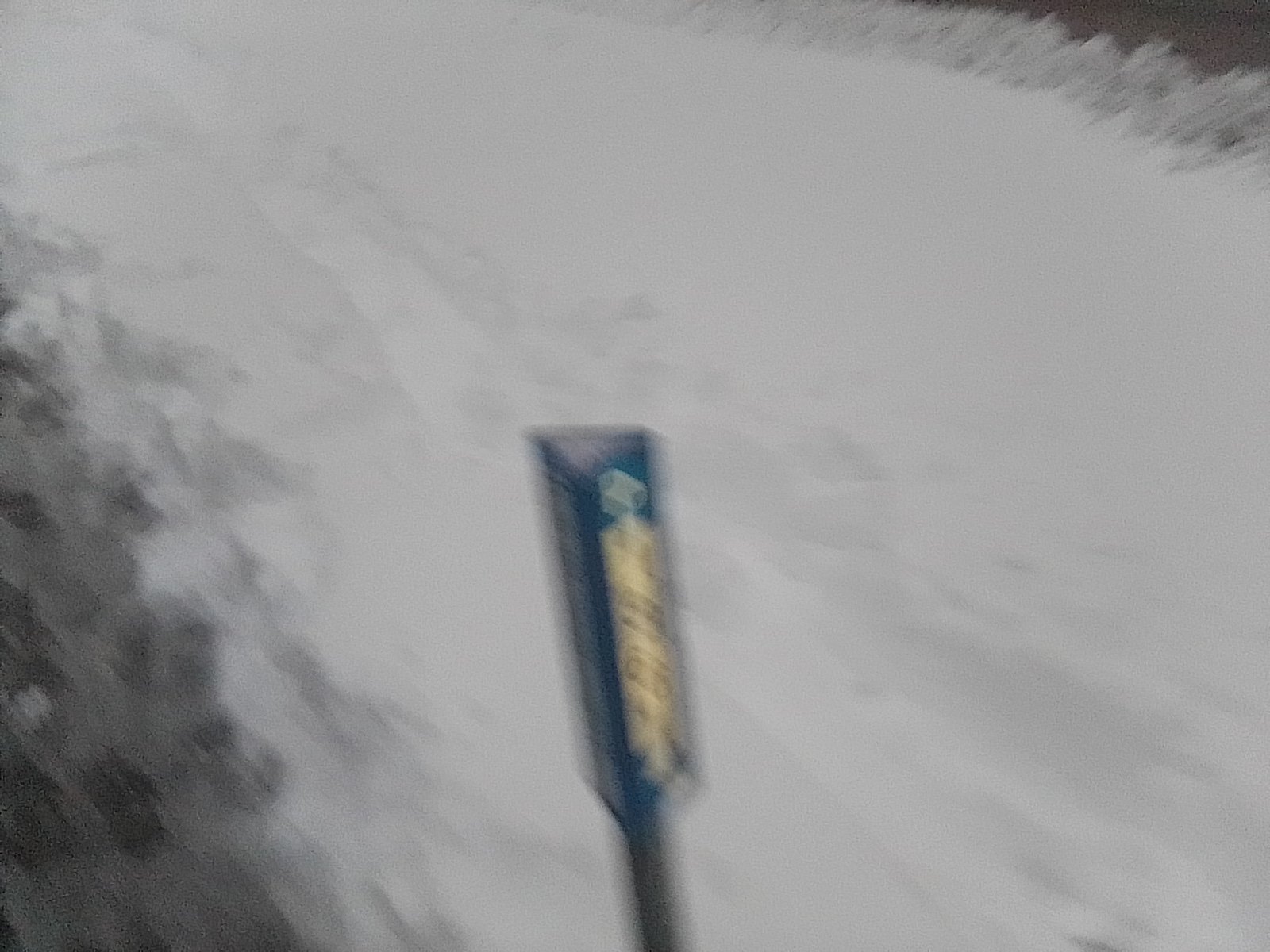In this exceptionally blurry and dimly lit photograph, we can make out a powdery white snow-covered road area, interspersed with light gray shadows. The most prominent feature is a blue triangular sign mounted on a pole, rising from the center of the image and extending to about half the photograph's height. The sign includes a white label or stripe along one side of the triangle. Flanking the road, both in the lower left and the upper right corners, are dark, indistinct forms that may be shrubs, trees, or another path. The overall graininess and poor lighting of the image make it challenging to discern further details.